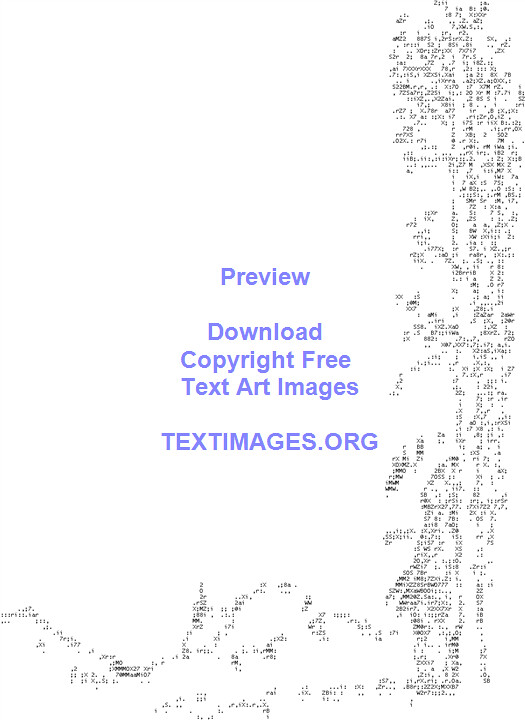The image showcases a form of text art, specifically ASCII art, where letters and numbers are meticulously arranged to create a drawing or sketch on a plain white background. Most of the black text is concentrated on the right-hand side and along the bottom of the image, forming an intricate, albeit chaotic, design that resembles someone standing next to a tree, with potential additional elements like ground or clouds. Due to the low resolution, the exact depiction remains unclear. Prominently, in the center of the image, there's muted purple text that reads "Preview Download Copyright-Free Text Art Images, textimages.org" with "textimages.org" in all capital letters.